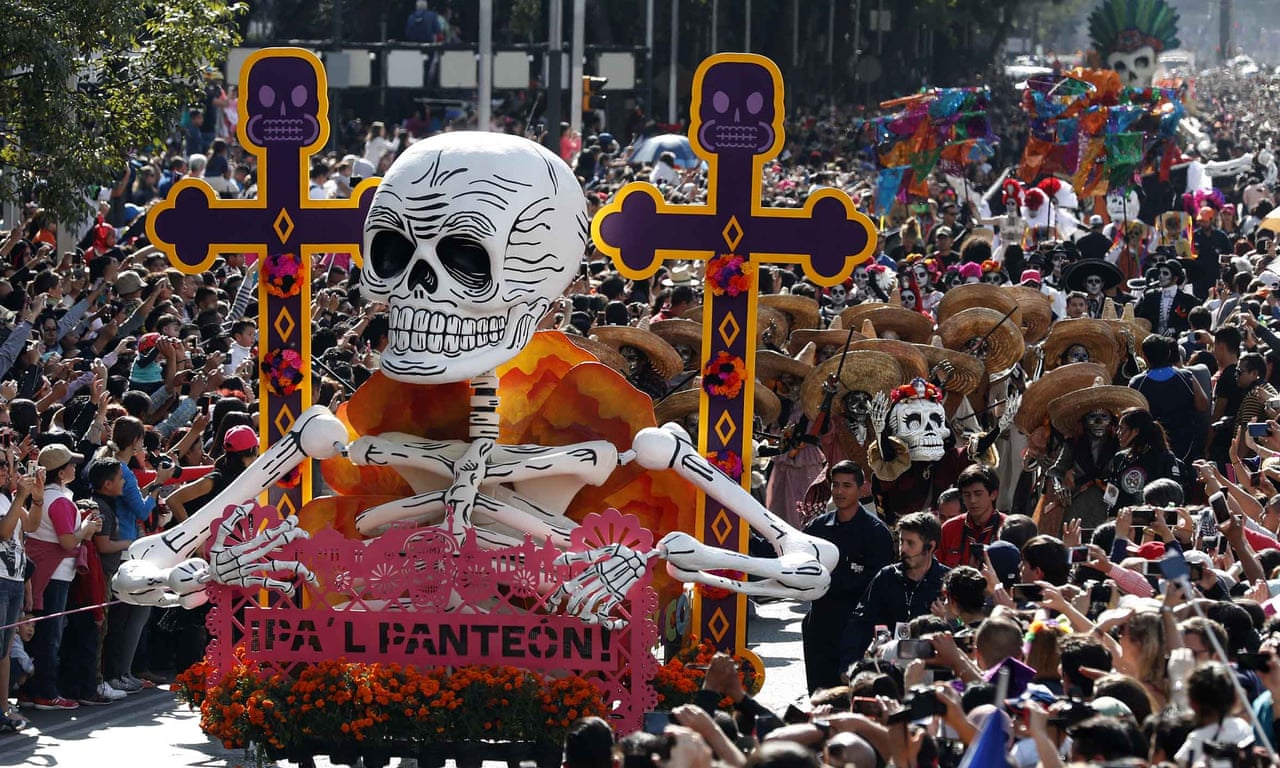The photograph captures a lively and colorful parade, possibly set in Mexico, celebrating the Day of the Dead. The streets are lined with a crowd of at least a thousand onlookers, many of whom are adorned with skull face paint and wearing large sombreros. The prominent float in the image features a giant, black and white skeleton seated amidst an array of flowers, with the inscription "Ipa la Pantellon." The float also displays black and gold crosses with diamond decorations, adding to the vivid atmosphere. In the background, another skull-themed float is visible in the upper right corner, and several other colorful floats fill the space in between. The parade, abundant with vibrant colors like blue, purple, pink, and orange, exudes joy and celebration, reflecting a festive commemoration of life and death. A couple of security personnel can be seen walking along the parade route, ensuring the crowd stays behind the roped-off area.